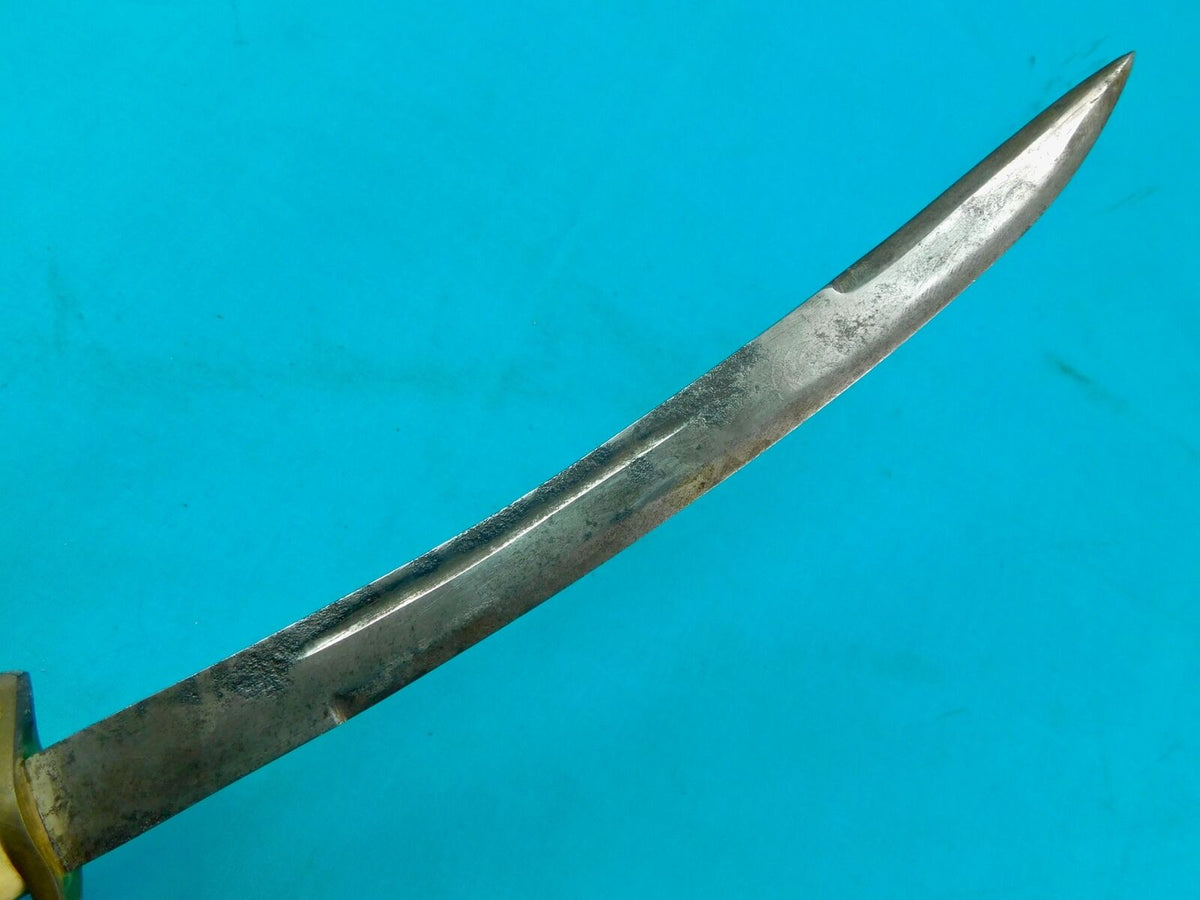The image is a large square with a blue background, reminiscent of the sky but marred by gray stains and streaks of darker shades. Dominating the scene is an old, antique sword, angled from the lower left to the upper right corner, culminating in a sharp tip pointing upward. The handle, barely visible in the lower left corner, is gold-colored but discolored with patches of green. The silver blade itself shows signs of extensive wear and oxidation, featuring blackened areas, especially in the middle, where a long indentation runs along its length. The top edge of the blade is smooth, contrasting with the bottom edge, which appears more eroded and rugged. The historical and weathered condition of the sword evokes a sense of age and storied past.